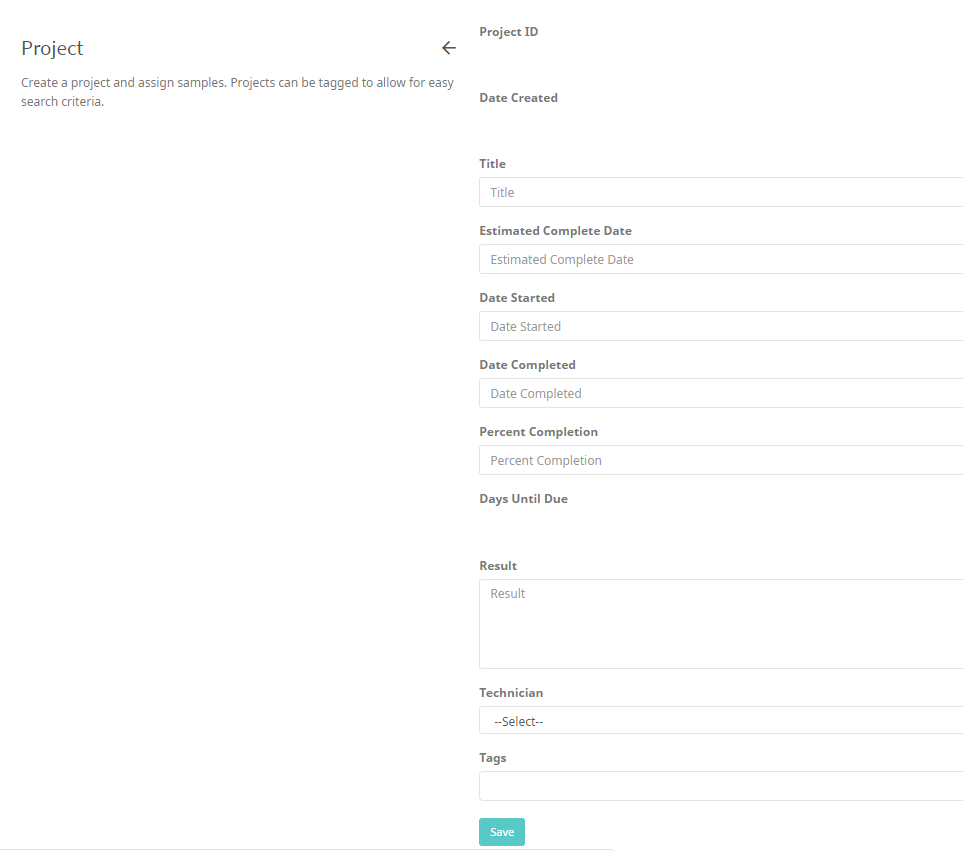The screenshot showcases a user interface (UI) in dark gray text with multiple input fields and informational labels for managing projects. 

In the upper left corner, a section titled "Project" is prominent. This area allows users to create a new project and assign various samples to it. Additionally, projects can be tagged to facilitate easy search through specific criteria.

On the right side of the image, there is a label "Project ID" accompanied by a left-pointing arrow. Underneath that, fields are provided for "Date Created" for recording the initial setup date of the project. Below these fields, there are several white input boxes with respective labels both inside and above each box. These inputs include:

- "Title"
- "Estimated Completion Date"
- "Date Started"
- "Date Completed"
- "Percent Completion"

Each of these boxes is meant to capture detailed project information.

Further down, there's a section labeled "Dates Until Due," followed by "Result." The "Result" section has a large box presumably to input detailed result descriptions pertaining to the project outcome. 

Beneath the result box, there is a "Technician" input field with a dropdown box that says "Select," indicating that the user can choose a technician associated with the project. Below that is a "Tags" box for inputting tags related to the project for better organization and retrieval.

Finally, at the bottom right, there is a blue action button labeled "Save" for saving the project details once all necessary information has been entered.